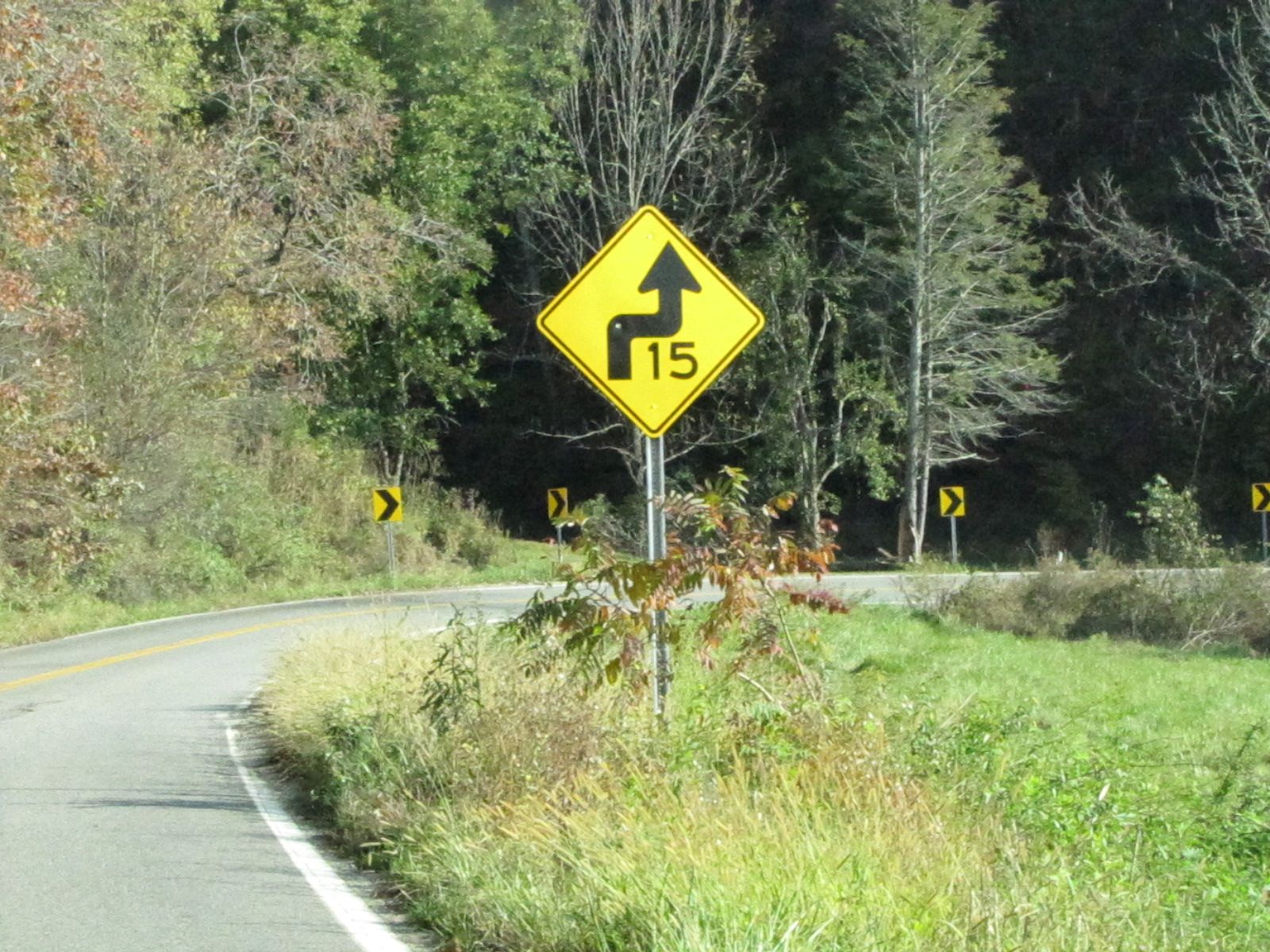The image depicts a serene outdoor scene featuring a winding road that curves to the right. The road itself is a classic black asphalt surface, adorned with a single yellow stripe running down the center and a white stripe along the right edge, guiding the way. To the right of the road, there's a patch of tall, unkempt grass.

Amidst the grass stands a road sign, nearly obscured by overgrown weeds and twigs with brown leaves. The sign is mounted on a silver metal post and features a bright yellow background with a bold, black numeral "15" at the center. It's outlined in black and also bears a large, thick black arrow that goes straight, curves sharply to the right, and then continues straight again, signaling an upcoming turn.

Along the road, smaller signs with yellow backgrounds and black arrows point straight ahead, serving as additional reminders of the road’s twists and turns. The background of the scene showcases a diverse array of trees, some of which are evergreens that maintain their verdant foliage year-round, while others display leaves in various states of seasonal transition—some changing colors, others barren with an autumnal dryness.

The left side of the image includes several large trees with leaves that appear dry and brown, hinting at the changing season. The sun casts a soft glow, its light creating reflections and shadows on the road, adding warmth to the peaceful roadside scene.